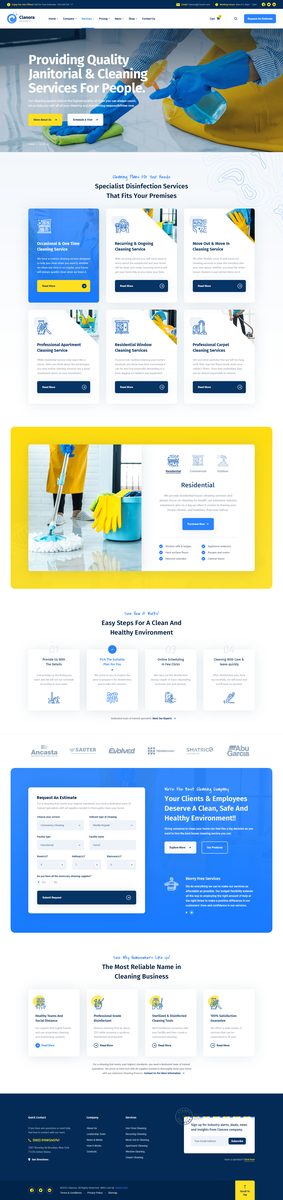The screenshot from the website is quite small and becomes blurry when enlarged, making it difficult to discern individual details clearly. Across the top, there is a very dark blue bar featuring several yellow icons and small inscriptions in white. Directly beneath this, there is a horizontal white bar. On the left side of the bar, a round blue and white logo is visible.

Below this logo, the website lists several sections, with one of them highlighted in blue, indicating it is currently selected; the rest of the text in this menu is in black. On the far right of the white bar, there is a blue button with white text.

Beneath this structure, a thicker banner spans the width of the page. This banner displays an image of a person wearing blue rubber gloves, using a green cloth to wipe a highly reflective, shiny white surface. Superimposed on this image is the prominent text: "Providing quality janitorial and cleaning services for people" in large white letters. Beneath this bold statement, there is smaller, unreadable text, followed by side-by-side yellow and white buttons.

Following the banner, six smaller boxes are arranged in two rows of three. Above these boxes is the phrase "Specialist disinfection services that fit your premises." Further down, a yellow box contains an image of a person mopping the floor with the caption "Residential" adjacent to it.

At the very bottom of the screenshot, a large blue box contains the text: "Your clients and employees deserve a clean, safe, healthy environment."